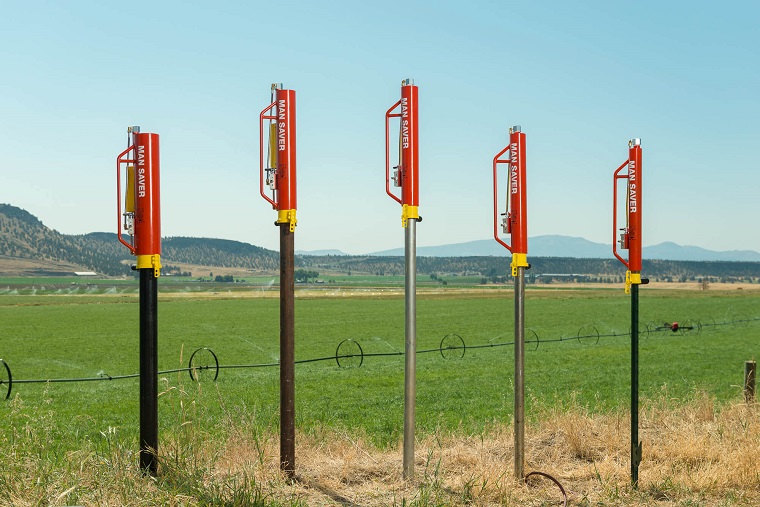This is a detailed photograph taken outdoors, showcasing a row of five poles erected in a ground area. The poles vary in color, including black, dark brown, and different shades of silver. They are cylindrical in shape and each has a device attached near the top, which is also largely cylindrical with a handle towards the left side. The devices are predominantly red and yellow, and feature text that reads "Man Saver." A barbed wire runs horizontally behind these poles. The ground beneath the poles appears slightly brownish, while the area beyond is covered in lush green grass. In the background, several hills, covered in dark trees, rise up against a clear blue sky with no clouds. The scene suggests a protective setup, possibly to guard a farm or similar area from predators.